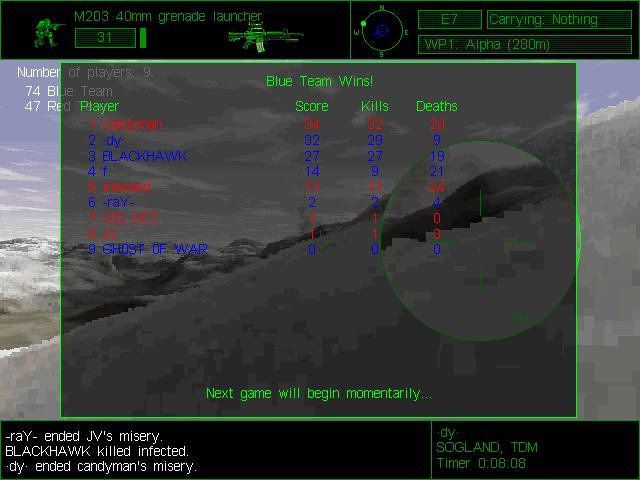The image is a detailed screenshot from a video game. The background features a scenic mountain range with a blue sky and scattered clouds, subtly visible through a grayed-out overlay. In the top left corner, "M203, 40mm grenade launcher" is displayed. On the far left, a crouched figure is holding a gun aimed forward. Just to the right, there is a vertical green rectangle with the number "31" inside, likely indicating ammo count.

To the right of the rifle icon, a compass shows directions (North, East, South, West) with a light gray dot marking a specific point. Further to the right, several rectangular icons display player stats: "E7" marks one, and another labeled "WP1 Alpha, 280mm" follows.

The interface also features a scoreboard showing detailed player statistics. The blue team, with 74 points, is declared the winner over the red team, which has 47 points. There are fields for each player's score, kills, and deaths. Notably, the bottom black border lists various in-game events and player actions in white text: "Ray ended JV's misery," "Blackhawk killed Infected," and "D.Y. ended Candyman's misery." Green text on the lower right reads, "D.Y. Sawgland Tom Timer 00808." Centered in the grayed-out box are the words "Blue Team Wins," and below it, "The next game will begin momentarily."